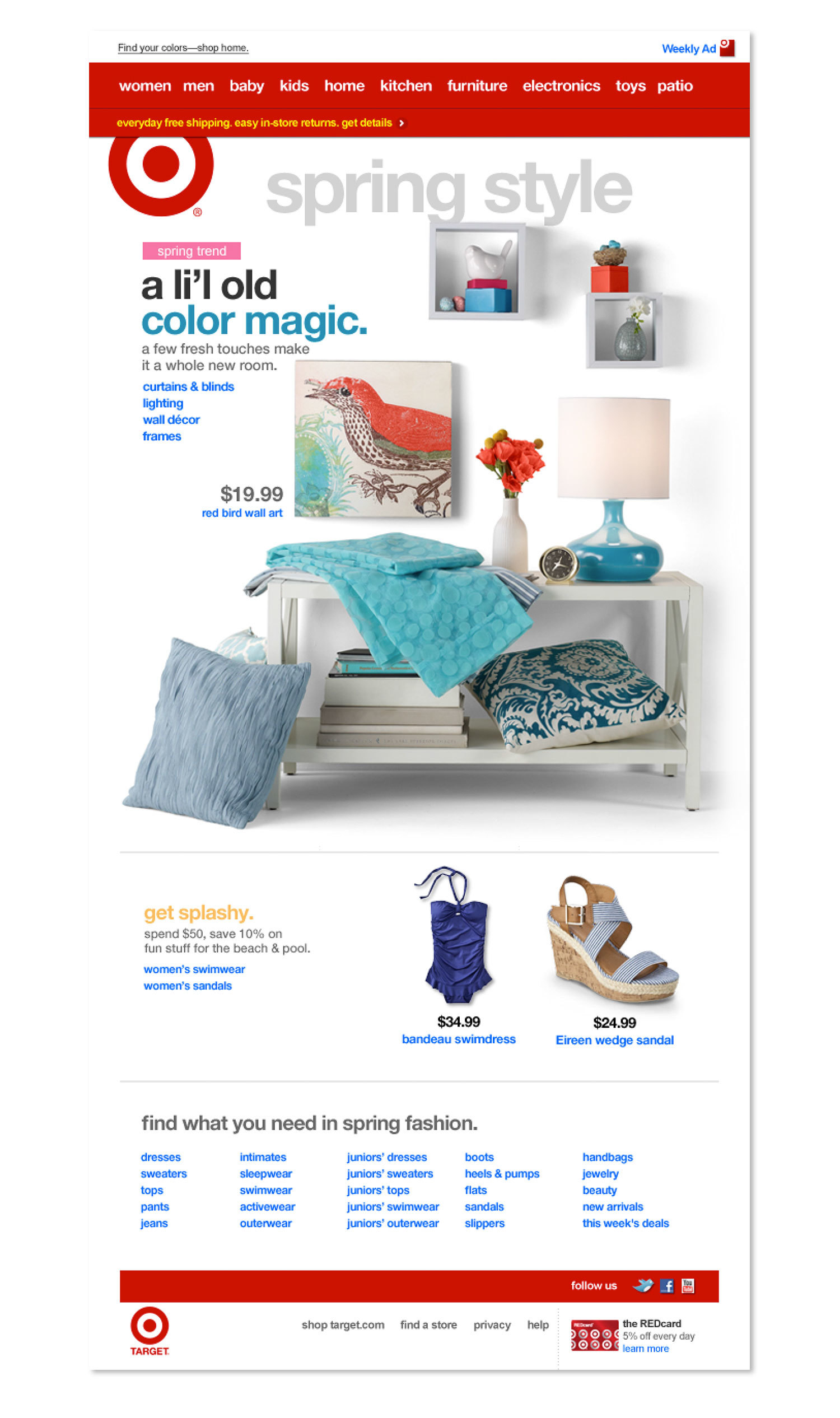The Target website homepage features a prominently placed Target logo in the top left corner. A horizontal navigation bar located above the logo offers various shopping categories such as Women, Men, Baby, Kids, Home, Kitchen, Furniture, Electronics, Toys, and Patio. An additional bar above this features offers like "Everyday Free Shipping," "Easy In-Store Returns," and more details.

Below the navigation, a large Target icon accompanied by the text "Spring Style" introduces the spring trends with the slogan "Spring Trend: A Little Old Color Magic. A Few Fresh Touches Make It a Whole New Room." This section highlights categories like curtains and blinds, lighting, wall decor, and frames. The featured example showcases a styled room with decorative pillows, wall art, a lamp, fresh flowers, and a small desk accessorized with books.

Further down, a promotional banner with the text "Get Splashy: Spend $50, Save 10% on Fun Stuff for the Beach and Pool" displays a colorful selection including a swim dress and sandals. This is followed by another section titled "Find What You Need in Spring Fashion," featuring clickable blue text links directing to various fashion categories.

At the bottom right corner of the page, the Target logo is shown again along with information about the Target RedCard.